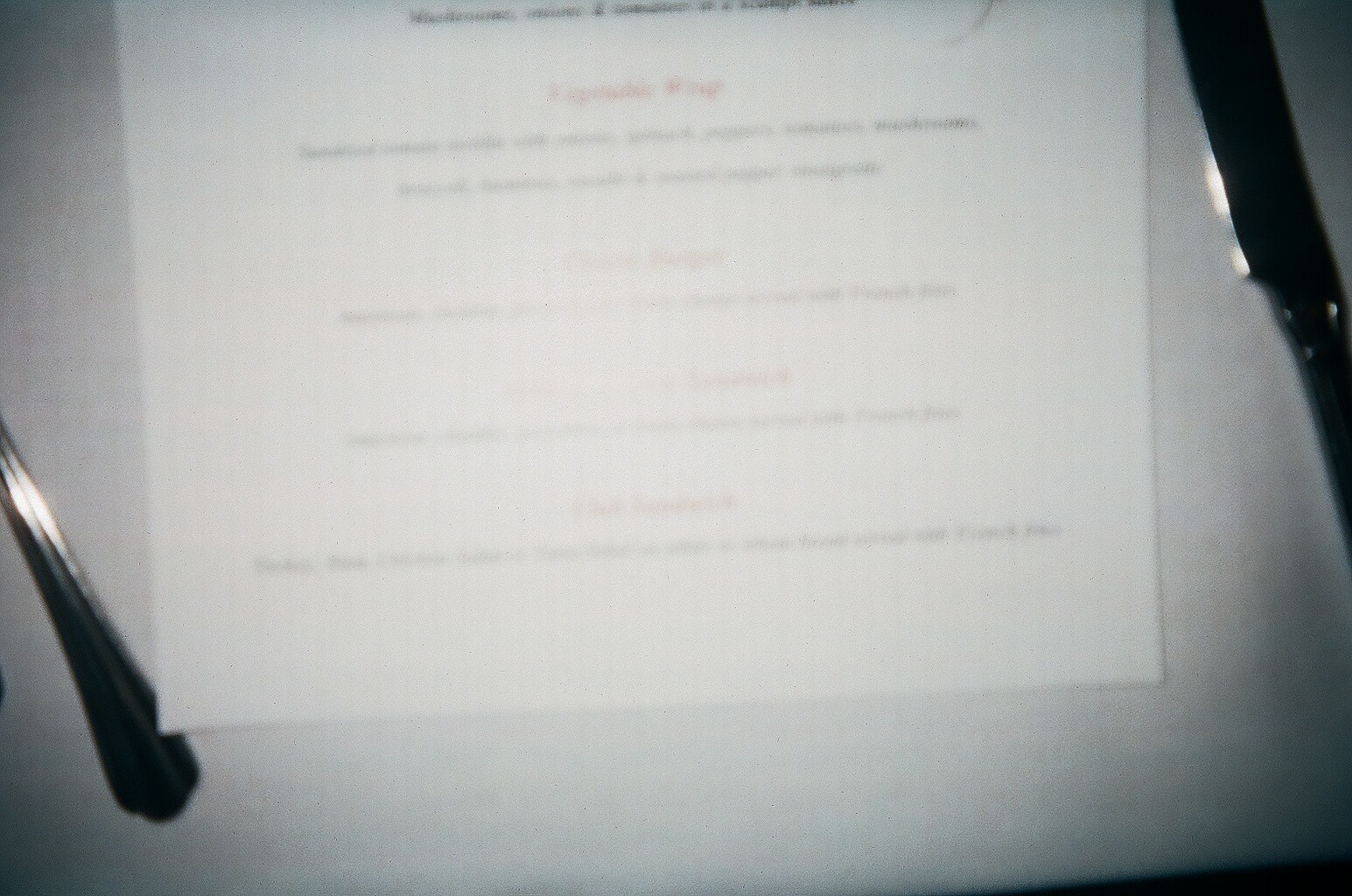A grainy black and white photograph depicts a scanned or photographed image of a piece of paper placed on a white table. The photo is taken from a top-down perspective and only half of the paper is visible. To the right, part of a butter knife is seen on the table. The tip of the knife is cut off at the top edge of the photograph, and the handle is truncated around the middle of the image, leaving only a portion of the blade and handle in view. In the bottom left corner, adjacent to the piece of paper, the handle of a piece of silverware is visible, angled towards the center of the left side of the image, although the type of utensil remains unclear as it extends out of the frame. The document on the table features a top line of dark black, bolded text, followed by some spacing, a red font header, a small segment of black text, another red header, and subsequent black text. This pattern is repeated two more times below.